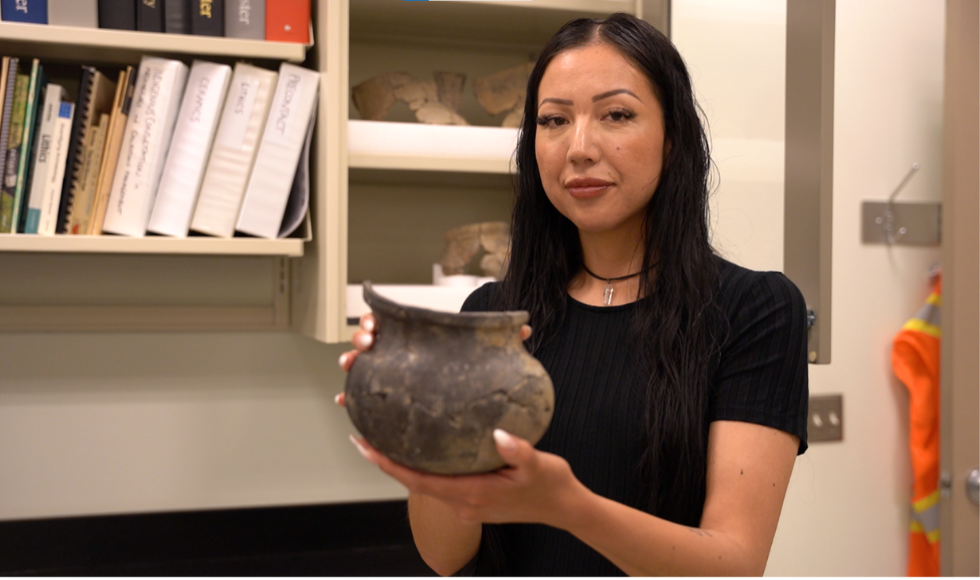This photograph captures a young Asian woman with long black hair parted in the middle, wearing a black t-shirt and a necklace featuring a black rope and a silver medallion. She is holding an old, handcrafted clay pot with a dark gray or black exterior and lighter brown patches. Her fingernails are painted white. The woman is standing in a well-lit office with white walls, looking directly at the camera. Behind her, there is a shelf organized with white binders, books, and notebooks. Some of the book titles are partially readable, including words like "ceramics," "logistics," and "McCloud." To her right, there is a collection of artifacts, possibly fossils, displayed on another shelf. In the bottom right corner, a vibrant orange safety vest with yellow and reflective gray bands is visible. Additionally, a metal plate with light switches is attached to the wall, and the room’s lights are on.